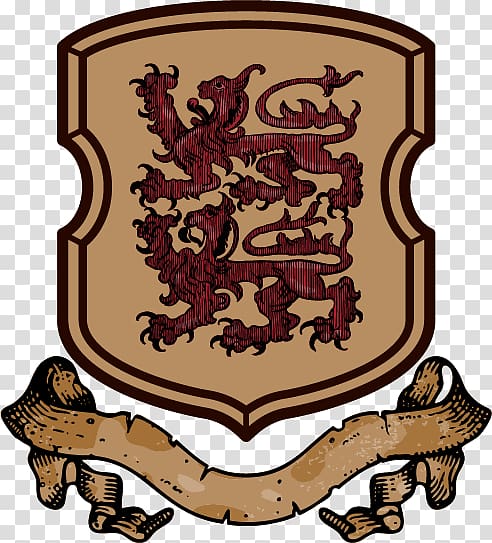The image is a detailed family coat of arms set against a checkerboard background of white and gray squares. The central element is a light brown, almost wood-colored shield, tapering to a point at the bottom. Flanking the sides of the shield, there are two intricate red dragons, reminiscent of old-timey or Tudor-style lions, stacked one above the other. Both dragons face left, each with its right paw extended upward. Beneath the shield, there's a ribbon or parchment scroll with vintage, tangled edges, intended for a family name or a Latin motto, though it remains blank in this illustration. This vector-like image, possibly a PNG file, is ready to be personalized according to the user's needs.